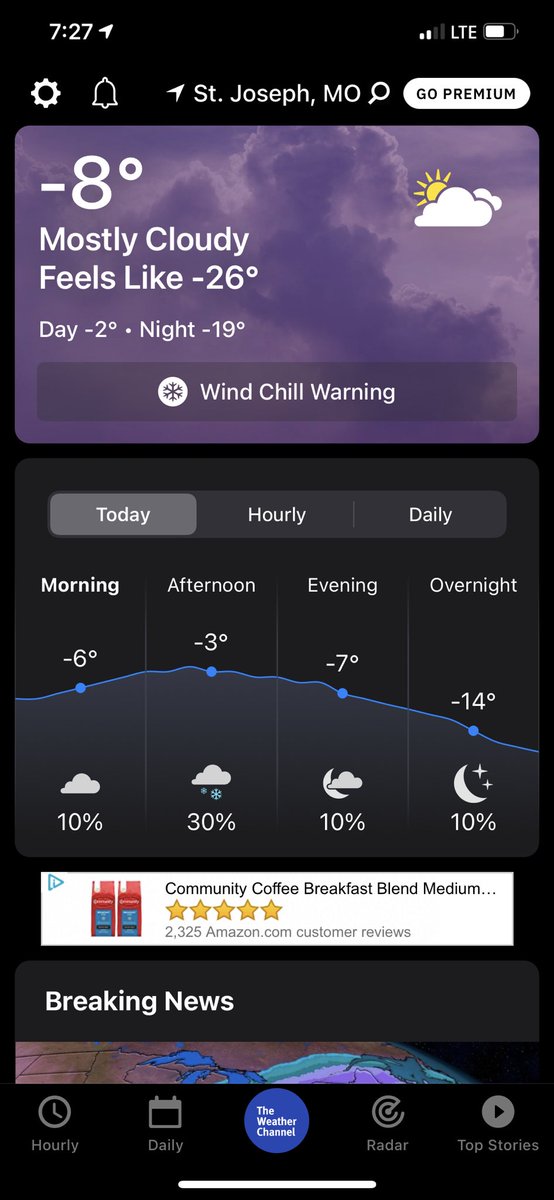A close-up image of a smartphone screen displaying a detailed weather forecast for St. Joseph, MO. At the top, the screen shows the time alongside a white location arrow, LTE signal, battery percentage, settings gear icon, and a notification bell. The header also includes icons for a magnifying glass, "GoPremium" button, and notes the current weather as mostly cloudy with a temperature of -8°F, feeling like -26°F. The daytime high is predicted to be -2°F, with a nighttime low of -19°F. A windchill warning accompanied by a snowflake icon is prominently displayed.

Below this, an hourly forecast for the day is presented, segmented into morning, afternoon, evening, and overnight. A blue line graph indicates temperature variations: -6°F in the morning with a 10% chance of precipitation, -3°F in the afternoon with a 30% chance, -7°F in the evening with a 10% chance, and -14°F overnight with another 10% chance.

The screen also features an advertisement and a breaking news section at the bottom. Navigation buttons for "Hourly," "Daily," "The Weather Channel," "Radar," and "Top Stories" are situated at the very bottom of the screen. The overall background is dark, with white text and a section showcasing a purple cloud. The meticulous detailing of the smartphone's display provides comprehensive weather information at a glance.